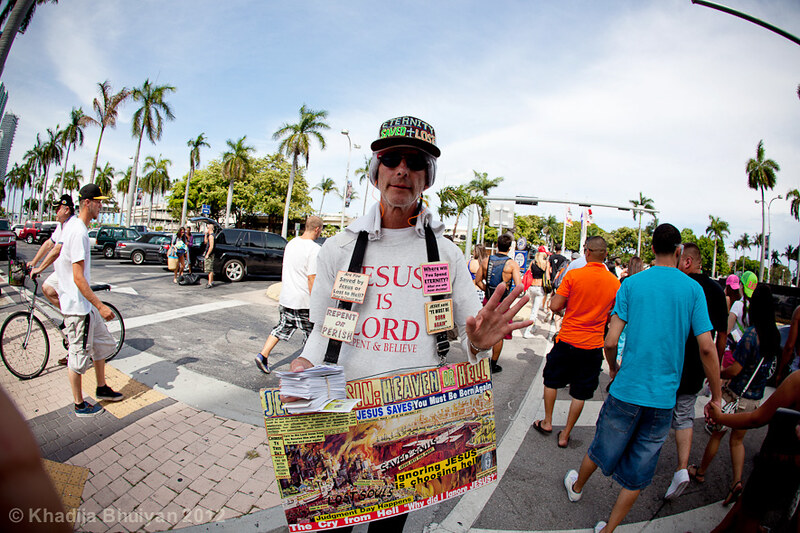In this horizontally aligned rectangular image, taken outside in a tropical setting, a man stands prominently at the center. The background is lush with many palm trees and other green-leaved trees, under a sky blanketed with thin white clouds. On the left side of the frame, a couple of people are visible—one standing and the other atop a bicycle. The right side shows numerous people, dressed in t-shirts and shorts, walking away from the viewer, seemingly crossing a road or parking lot.

The focal point of the image is an older white man with gray hair peeking from underneath a black hat, which reads "eternity saved and lost." He wears black sunglasses and a white long-sleeved shirt emblazoned in red text: "Jesus is Lord, repent and believe." Around his neck is a large, colorful rectangular sign with black straps, filled with messages about Jesus, heaven, and hell. The sign bears phrases like "ignoring Jesus is choosing hell" alongside graphic depictions. In his left hand, he waves towards the camera, while his right hand holds a bundle of papers or index cards bound by a rubber band. The photograph, shot with a fisheye lens, captures this man's fervent street-side protest in vivid detail, emphasizing his passionate display of religious warnings. In the bottom left-hand corner, the image credits photographer Khadija Boyan, dated 2012.